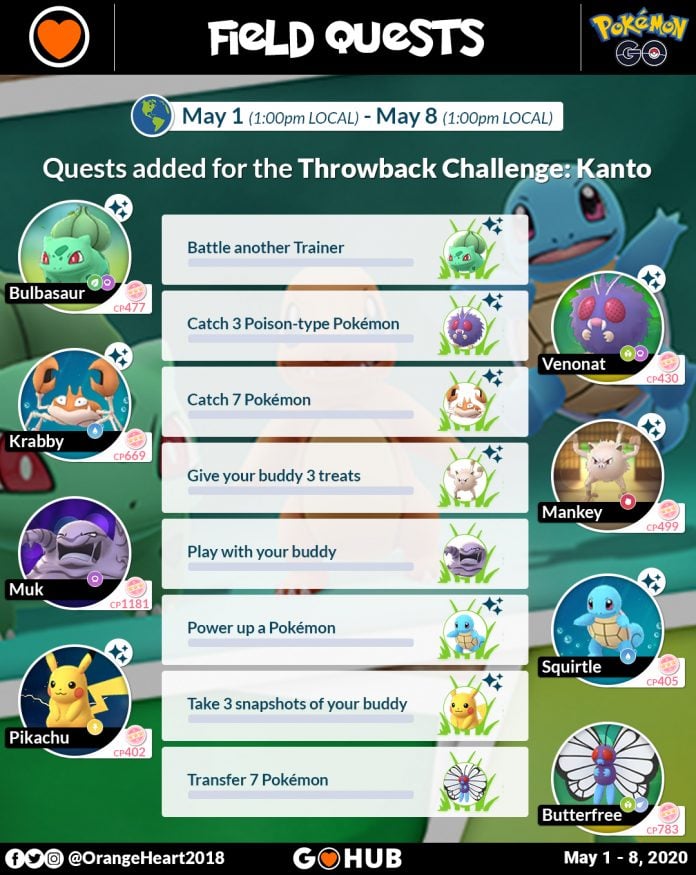The image is a detailed chart from the Pokémon GO Throwback Challenge event running from May 1st to May 8th, starting at 1:00 PM local time. At the top of the chart, there's a prominent red heart enclosed within a white circle, symbolizing the event's theme. Located centrally at the top, the heading "Field Quest" is written in white. Below this, the iconic "Pokémon GO" logo appears, with "Pokémon" in yellow and "GO" underneath it.

The chart includes a quest announcement, specifying the event as the "Throwback Challenge: Kanto." The image is divided into sections, with eight Pokémon characters featured prominently. On the left side, the characters listed are Bulbasaur, Krabby, Murkrow, and Pikachu. On the right side, the characters are Venonat, Mankey, Squirtle, and Butterfree.

In the central column of the chart, there's a list of tasks participants need to complete, including:
- Battle another trainer
- Catch three Poison-type Pokémon
- Catch seven Pokémon
- Give your buddy three treats

This detailed chart offers a clear overview of the event's schedule, featured Pokémon, and specific tasks required to complete the Throwback Challenge.